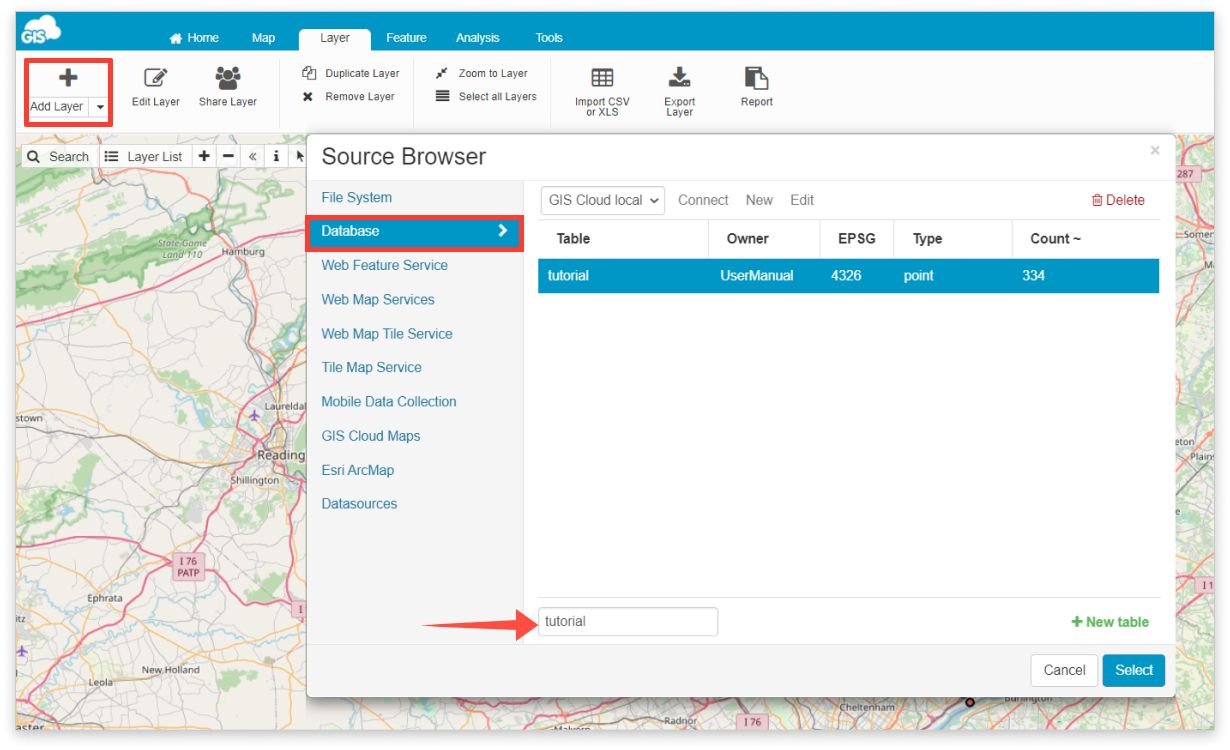A detailed screenshot of a GIS (Geographic Information System) map website interface. In the upper left-hand corner, the logo "GIS" is prominently displayed in white text with a blue outline, accompanied by a cloud icon. The top of the web page features a blue navigation bar with six categories: Home, Map, Layer, Feature, Analysis, and Tools—where the "Layer" category is highlighted.

Below this, a horizontal white bar spans from left to right, featuring eight different categories. The first category, "Add Layer," is highlighted with a red square and includes a drop-down menu with a plus icon. Following categories include "Edit Layer" with an icon, "Share Layer" with people icons, "Duplicate Layer," and "Remove Layer." Additional options in the bar are "Zoom to Layer" and "Select All Layers." Further along, there are options for "Import (CSV or XLS)," "Export Layer," and "Report."

In the background, the right-hand side of the screenshot reveals only a small portion of a detailed map displaying various locations in Pennsylvania. Key locations on the map include Hamburg, Reading, Shillington, New Holland, and the state game land park. A road marked as I-76 P.A.T.P. is also visible. At the bottom right, areas labeled Cheltenham and Radnor are noted.

Additionally, there is an inset white box titled "Source Browser," listing various data sources such as File System, Database, Web Feature Service, Web Map Services, Web Map Tile Service, Tile Map Service, Mobile Data Collection, GIS, Cloud Maps, ESRI, ArcMap, and others. The "Database" option is highlighted with a blue bar and a red outline. A red arrow points to the word "tutorial" inside a square search box.

The inset features a table with the headings: Owner, EPSG, Type, and Count. A blue row in the table is labeled "Tutorial Table," with the owner as "User Manual," EPSG code "4326," type as "Point," and count as "334." At the bottom right of the inset box, selectable options include "Cancel" or "Select."

Overall, the screenshot showcases a comprehensive and feature-rich GIS interface with multiple options for managing and analyzing map layers and data sources.